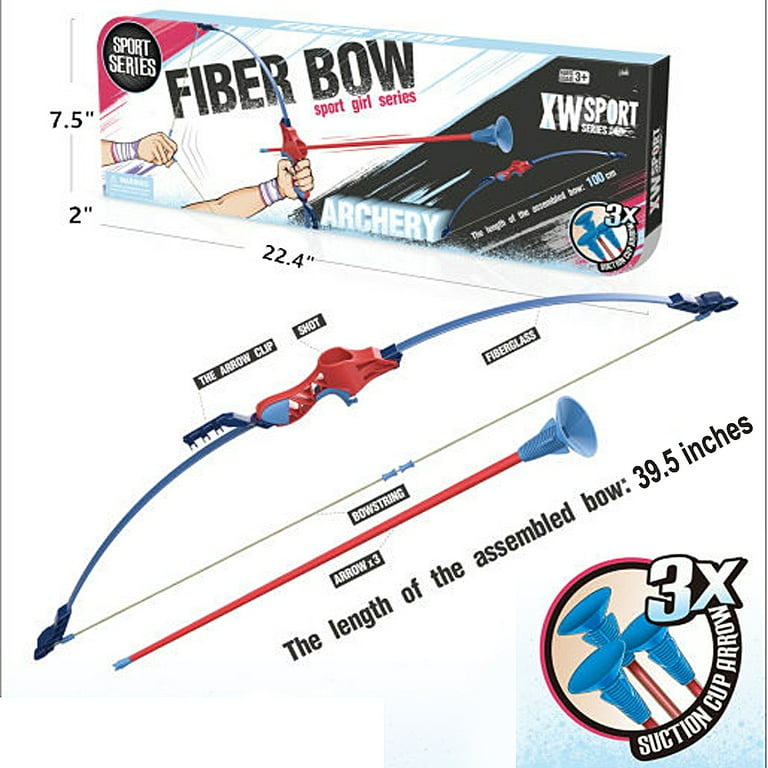This image is an advertisement for the Fiber Bow Sports Girl Series featuring a detailed layout of the product and its packaging. At the top, the box prominently displays the name "Fiber Bow" in black, with "Sports Girl Series" written in red. To the left, within a red patch, "Sports Series" is highlighted in white. A drawing depicts a person pulling back a bowstring with a suction cup arrow. On the right, against a black background, "Archery XW Sports Series" is written in white with a blue shadow. Below that, the size specifications are listed: 7.5 inches high by 22.4 inches wide.

Central to the image is the assembled bow, featuring a red handle and a blue bowstring. Above the bow, labels identify key components: the arrow clip, short fiberglass sections, and the bowstring. To the right of the bow, text states the assembled length as 39.5 inches. The bow is accompanied by red arrows with blue suction cup tips.

In the bottom right corner, a logo consists of three suction cup arrows arranged within a circle, surrounded by the text "3X Suction Cup Arrow." This logo is encased in a gradient blue-to-white square. The major colors in the advertisement—red, black, blue, and white—create a visually appealing design that highlights the product's features and specifications.